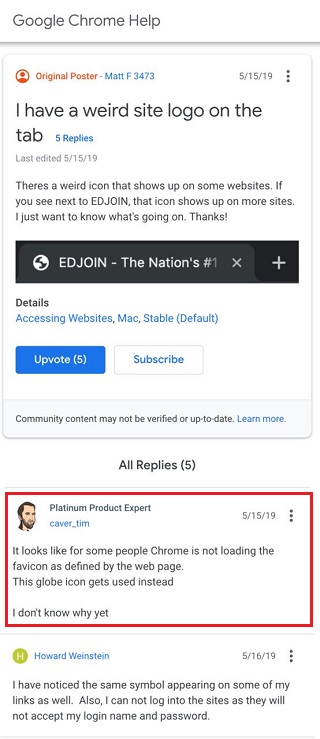The image depicts a forum post about a favicon issue on Google Chrome, displayed against a white background. The title "Google Chrome Help" is prominently featured at the top, followed by details of the original post and its replies. The post from May 5, 2019, includes the username "Original Poster" highlighted in red and "Mac F 3473" in blue, indicating a subsequent response. The main post reports an unusual site logo that appears as a favicon on certain websites, a concern echoed by a list of five replies marked in blue.

The post notes its last edit date as May 15, 2019. It discusses the appearance of a strange icon labeled "Join" on several websites, expressing a desire for clarity on the phenomenon. The writer indicates "Mac Stable (Default)" settings were in use while experiencing these issues. 

Below the post is a blue rectangle with "Upvote" in white text, the number five, and a blue "Subscribe" button. A gray rectangle provides a disclaimer: "This community content may not be verified or up to date. Learn more." It highlights that there are five replies in total. 

A detailed profile picture appears within another rectangle, identifying the user as a "Platinum Product Expert." The user's contribution is timestamped May 15, 2019, with an additional menu represented by three vertical dots next to it. The expert's commentary notes that Google Chrome sometimes fails to load the favicon as defined by the webpage, resonating with the original issue reported.